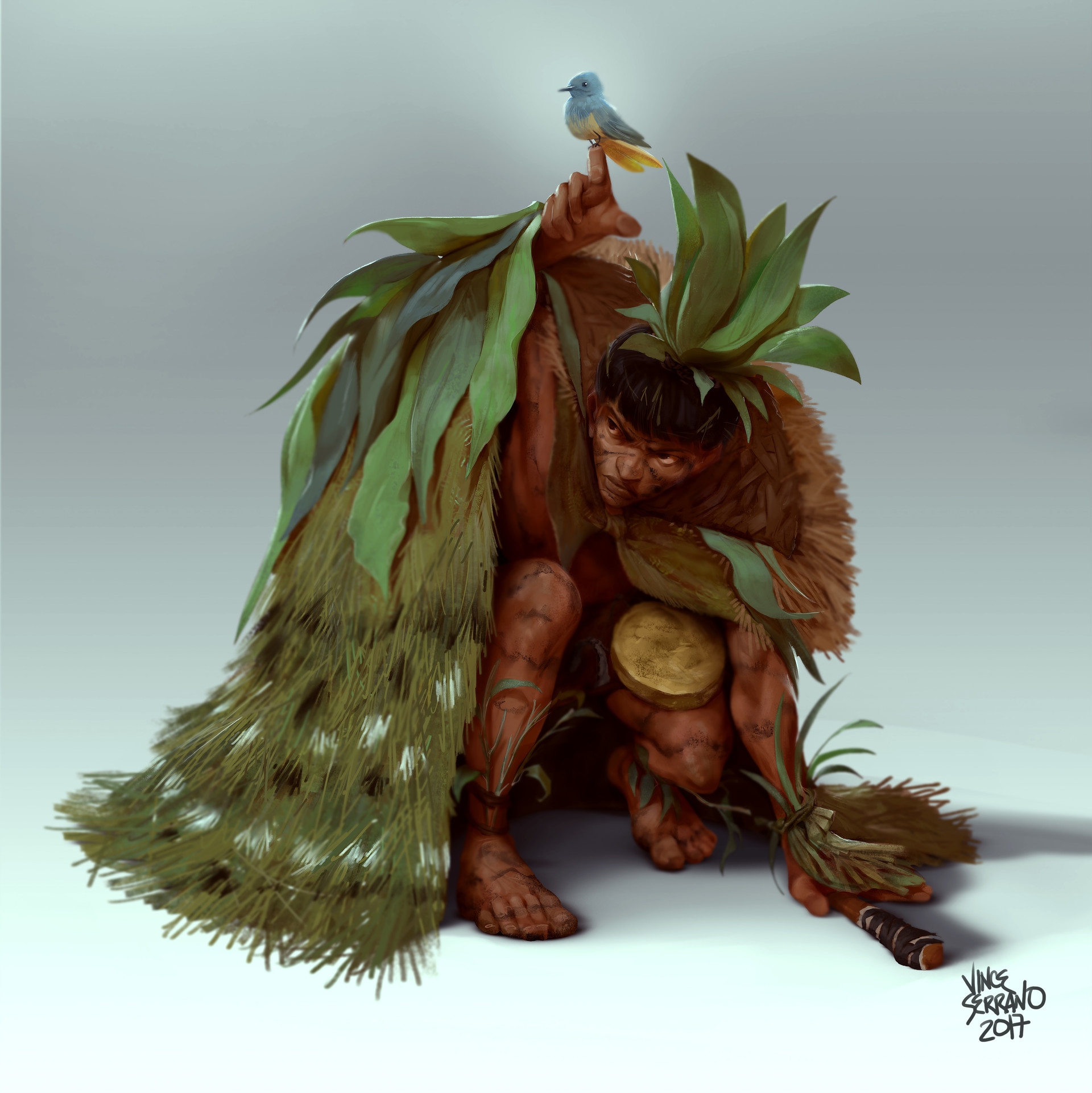In a digitally animated, square-sized image with a smooth style, a brown-skinned man resembling a caveman is depicted squatting or huddled towards the ground on a white floor, against a greenish background. The man is dressed in a cloak or cape made of grass, and palm leaves adorn his head and upper back, resembling a tree or indigenous attire. He holds an axe-like wooden tool in his left hand, which is resting on the ground, while his right hand is extended upwards, with a blue bird with a yellow tail perched on his index finger. A round yellow object, possibly a canteen, rests on his left knee. The scene casts a shadow extending to the right. The artwork is signed by the artist Vince Serrano, dated 2017.